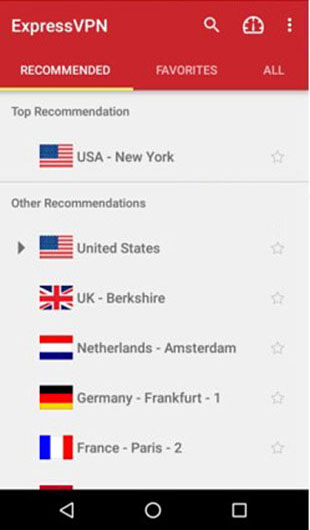This screenshot of the ExpressVPN interface showcases three tabs labeled "Recommended," "Favorites," and "All." The "Recommended" tab is currently selected. The interface prominently features a section titled "Top Recommendations," with a list of recommended server locations. 

- **Top Recommendations:**
  - **United States, New York** — Accompanied by the American flag.
  - **United Kingdom, Berkshire** — Accompanied by the UK flag.
  - **Netherlands, Amsterdam** — Accompanied by the Netherlands flag.
  - **Germany, Frankfurt** — Accompanied by the German flag.
  - **France** — Accompanied by the French flag.

The background of the Titles and Tabs is rendered in red, adding a bold visual emphasis. The flags and names of the countries are presented against a gray background, enhancing legibility. 

At the bottom of the interface, there are three symbols prominently displayed on a black background: a triangle, a circle, and a square, which may serve as navigational or functional buttons within the app.